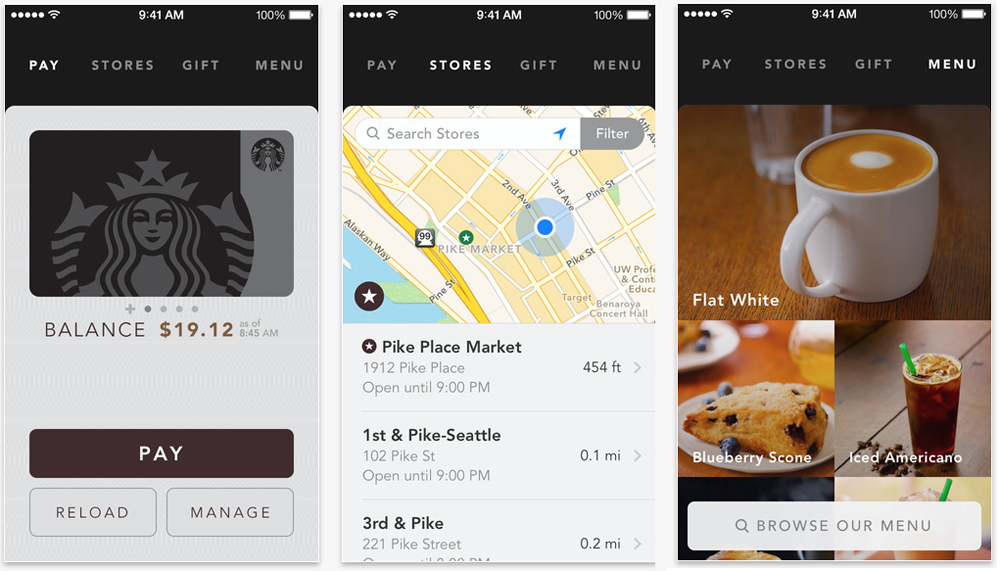This image is a collage of three smartphone screenshots displaying different pages of the Starbucks app. All three screenshots share a consistent design, featuring a black header with white text where the time is fixed at 9:41 AM. The app’s navigation menu, found at the bottom of each screenshot, includes options labeled "Pay," "Stores," "Gifts," and "Menu."

The central screenshot highlights the "Stores" page, displaying a map interface reminiscent of Google Maps, with markers for various store locations. This map is set in an unspecified city, but the presence of store listings named "First and Pike," "Pike Place," and "Third and Pike" indicates that the city is likely Seattle. Below the map, three store listings provide further details.

The right screenshot delves into specific menu offerings, showcasing three images: at the top is a steaming latte in a white cup, below it on the left is a photo of a blueberry scone, and on the lower right is a tall, chilled glass labeled "Iced Americano."

The left screenshot presents account details with the Starbucks logo in gray. Below the logo, the app displays a balance of "$19.12," and at the bottom, a prominent dark gray rectangular button with "Pay" inscribed in white font invites users to make a payment.

This detailed collection of screenshots offers a comprehensive look at various functionalities and features of the Starbucks app, from store locations to menu items and payment options.